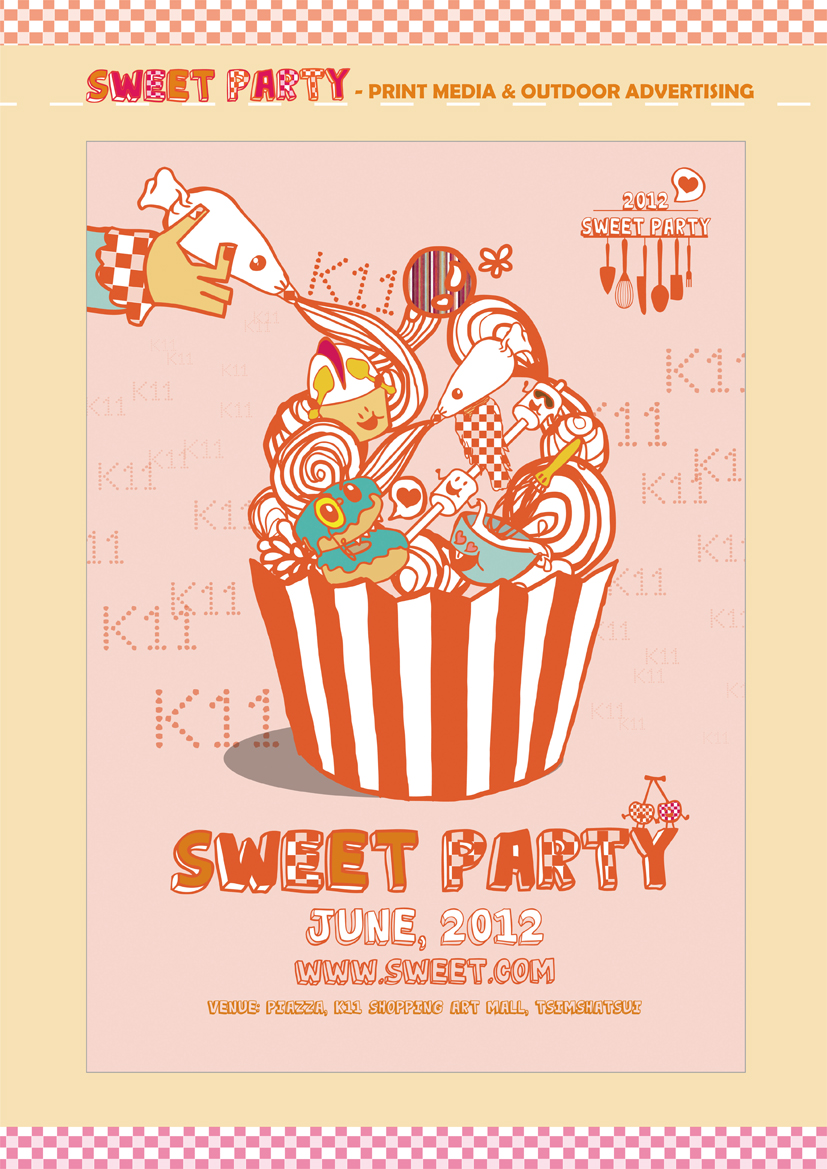This image appears to be a vibrant advertisement or invitation with an overall pink and light brown color scheme, accented by a pink checker pattern border at the top and bottom. The header, designed in colorful, cartoony text resembling candy wrappers, reads "Sweet Party" along with "print media and outdoor advertising." The central illustration showcases a whimsical scene of a cupcake being iced by a geometric hand. The cupcake is populated with animated, anthropomorphic characters like marshmallows wearing sunglasses, a living donut, and a mixing bowl with heart eyes. Surrounding the main image are repeating "K" and "11" symbols. Additional details include the text "2012 Sweet Party" in the top right corner and information at the bottom: "Sweet Party June 2012, www.sweet.com, venue: Piazza, K-11 Shopping Art Mall, Tsim Sha Tsui," all set against a lively backdrop of pink with yellow elements.